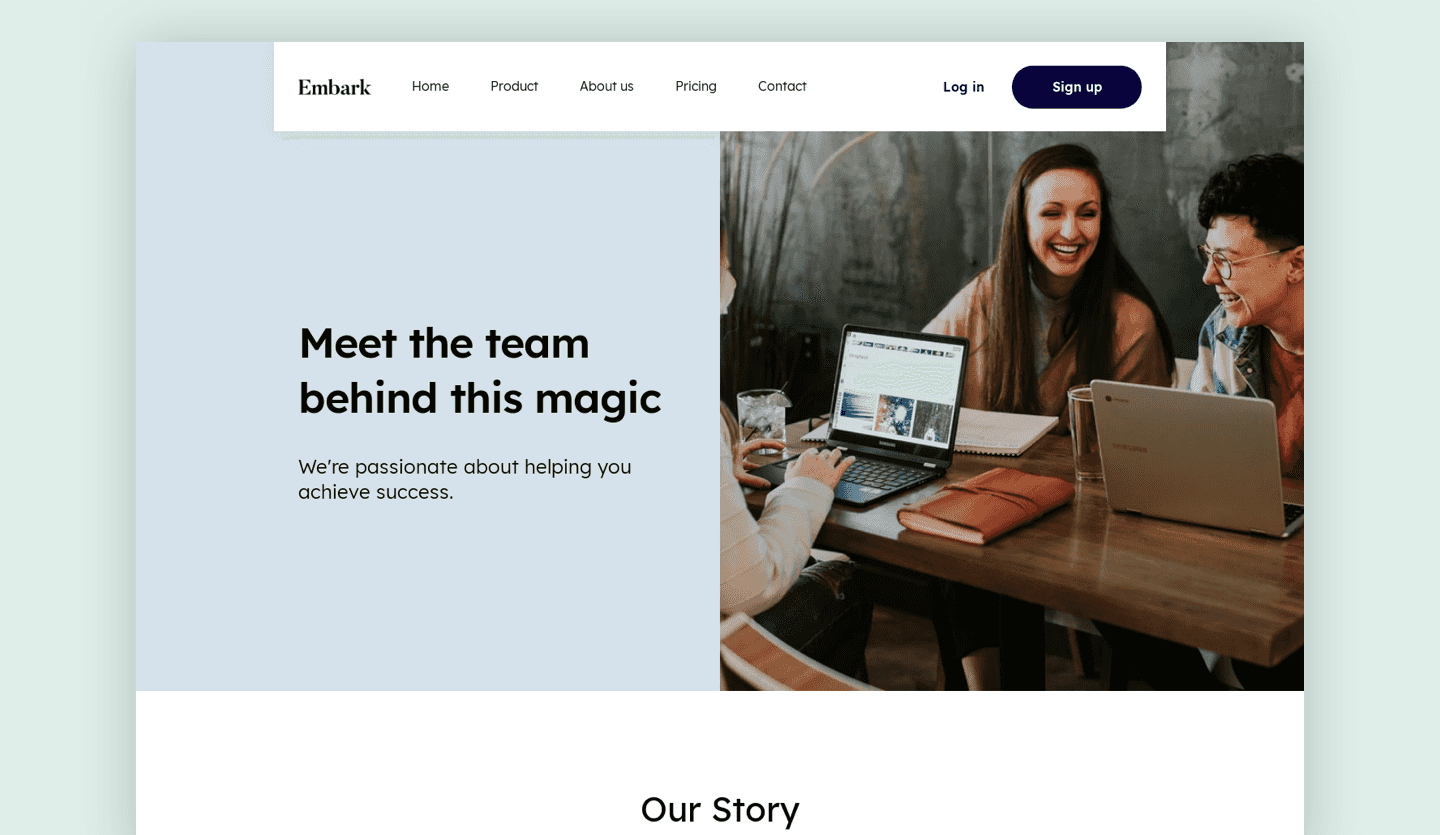This image is a detailed mock-up of a webpage from a website called "Embark." The composition features a large color photo on the right side, showing three people sitting at what resembles a picnic table, with an exposed concrete wall behind them. In the photo, two women are positioned with their backs to the wall, facing the camera; the one on the right has short hair and the one on the left has long hair, both laughing. The woman on the right has an open laptop in front of her. On the left edge of the photo, another woman is partially visible with a laptop screen facing her.

To the left of the photo, there is a gray text field containing a message: "Meet the team behind the magic. We're passionate about helping you achieve success." Below this text field, a white panel is labeled "Our Story."

The background of this entire section is a light mint color with a prominent drop shadow effect, giving it a layered appearance. At the top, spanning nearly 80% of the width, is a white rectangle that features the "Embark" logo on the left. Next to the logo, there is a menu bar with options such as "Home," "Product," "About Us," "Pricing," and "Contact." On the right side of this white rectangle, there are options for "Login" and a capsule-shaped blue button labeled "Sign Up."

This mock-up could be a template for sale or a work in progress for an actual company named Embark. The design is clean and organized, aimed at showcasing the company's team and mission effectively.